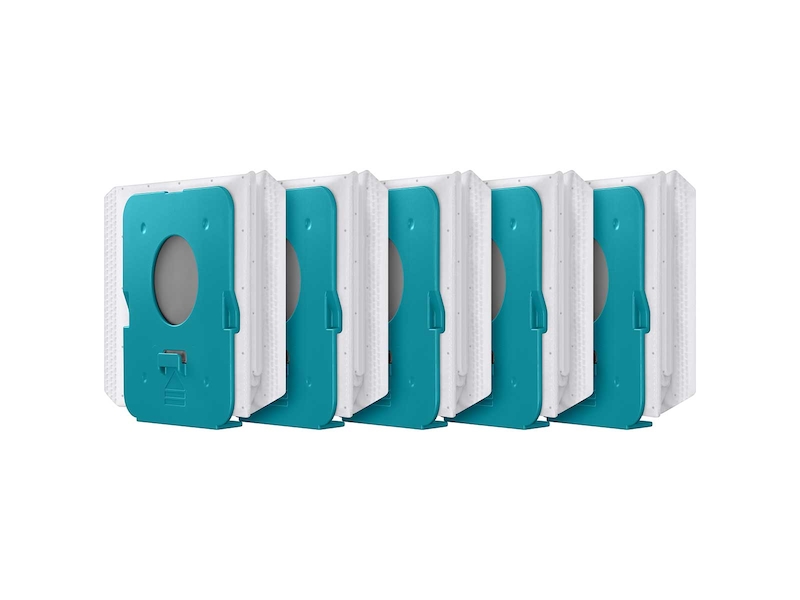This image features a set of five identical plastic holders, each containing folded white napkins. Set against a plain white background with no visible borders, these holders are arranged side by side, with some positioned slightly behind others, causing only parts of them to be fully visible. The holders are rectangular with a sturdy base plate that allows them to stand upright. 

Each holder has a distinctive design, featuring a turquoise-green rectangular panel with beveled edges on the front, made of plastic. In the center of this panel, there is an oval cut-out. Below the turquoise section, the design transitions to a grayish-toned area. At the bottom of each turquoise panel, there is an engraving of an upwards arrow.

The napkins within the holders are neatly folded, adorned with a dotted pattern. The combination of the holders' structural details and the positioning in the image emphasizes both their functional design as napkin holders and their aesthetic appeal.